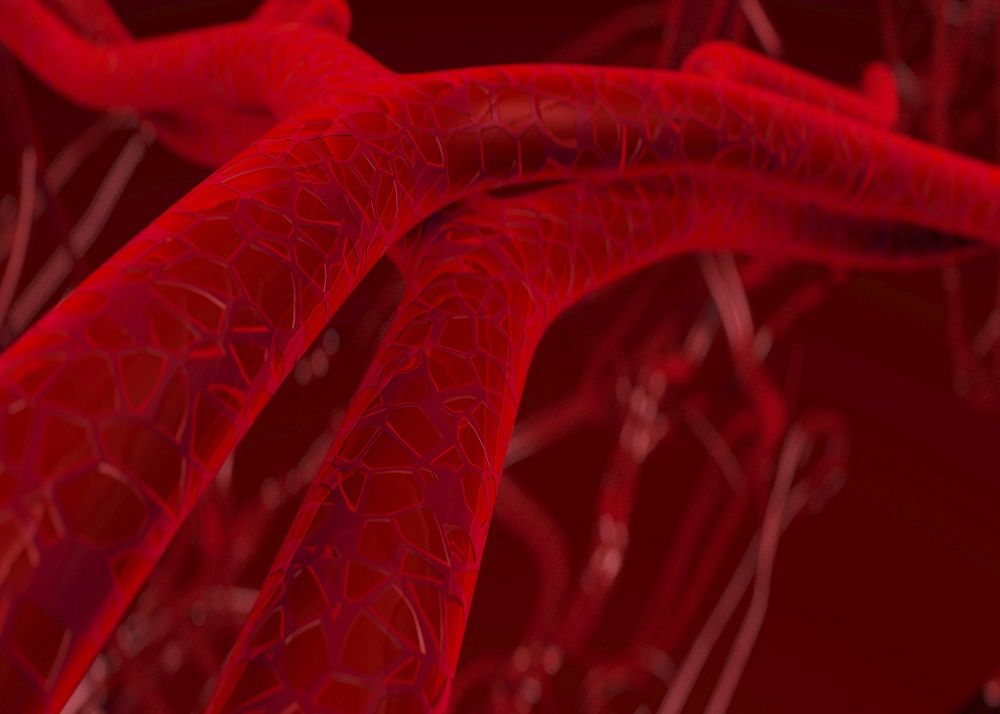The image is a highly detailed, computer-generated depiction that resembles the interior of the human body's vascular system. Dominated by a rich, blood-red color palette, the scene showcases two prominent arteries or veins originating from the bottom left and ascending towards the top middle before branching out in a Y-formation to the left and right. These main vessels exhibit intricate lines and striations on their surfaces, adding texture and realism. In the background, smaller, blurry vessels wind and twist in various directions, creating a complex and immersive network. The entire image, devoid of text, captures the essence of blood vessels streaming through the body, with some dark gray hues subtly appearing at the very top, further enhancing the depth and contrast of the composition.